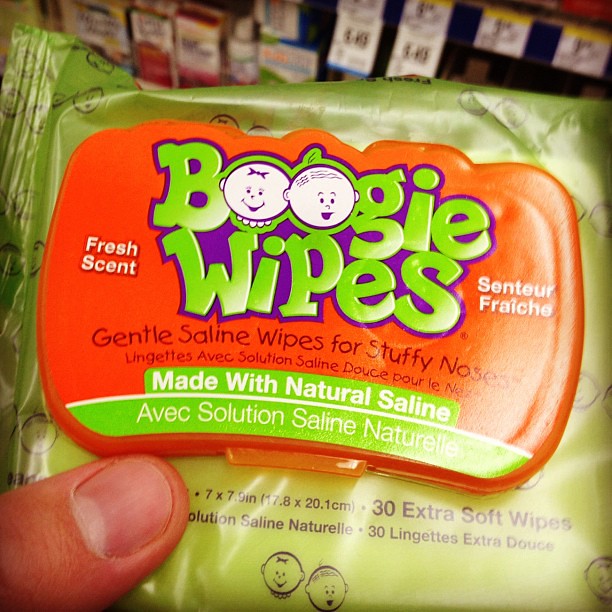The image features a person holding a packet of Boogie Wipes, identifiable only by their thumb. The packet is primarily lime green with an orange pattern on the front, and it has purple accents. The prominent Boogie Wipes logo is written in green text outlined in purple. Below the logo, the label reads "Gentle Saline Wipes for Stuffy Noses," with a bilingual note "Lingettes Avec Solution Saline Douce." The packet highlights its fresh scent and mentions that it is “Made with Natural Saline." Additionally, it specifies the quantity and size of the wipes: "30 Extra Soft Wipes" measuring 7 by 7.9 inches (17.8 by 20.1 cm). The label also includes illustrations of a boy and a girl, indicating that these are baby wipes. In the blurred background, there appear to be boxes of cough drops or cough medicine.